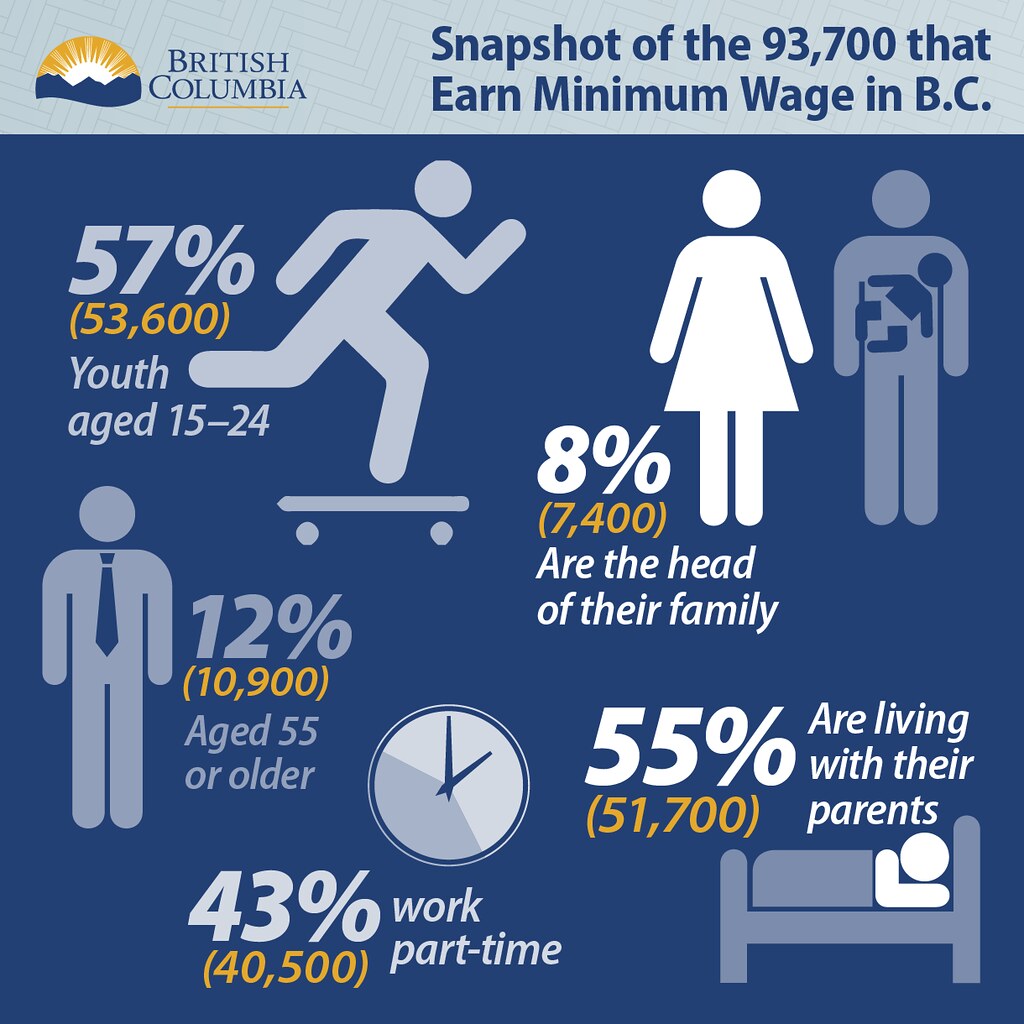The image depicts an infographic poster for British Columbia titled "Snapshot of the 93,700 that Earned Minimum Wage in BC." The poster features a blue background with well-spaced sections detailing various statistics. On the top left, there is a "British Columbia" logo with a sun and mountains, followed by the title. The main data points are illustrated with icons: 

- 57% (52,600 people) of minimum wage earners are youth aged 15 to 24, represented by a person on a skateboard.
- 8% (7,400 people) are the heads of their families, symbolized by a woman in a dress and a man holding a baby.
- 12% (10,900 people) are aged 55 or older, shown by a man in a suit and tie.
- 43% (40,500 people) work part-time, indicated by a clock.
- 55% (51,700 people) live with their parents, signified by a person lying in a bed.

The colors used are light blue, dark blue, white, yellow, and gray, contributing to the clear and accessible presentation of the data.